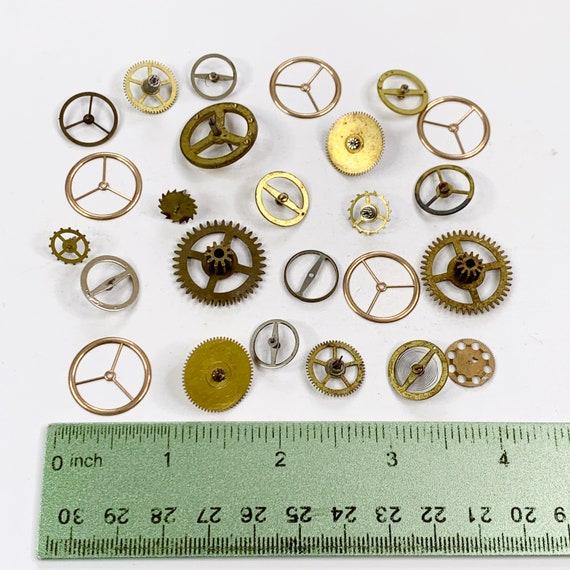The image features a variety of small, intricate metal gears and circular objects, resembling those found in watches and clocks, arranged against a white background. These pieces vary in size, none exceeding an inch, with the majority measuring around half an inch to three-quarters of an inch. The gears come in different colors, including bronze, gold, copper, silver, and black, with some displaying smooth edges and others showing cogs or rough patterns. At the bottom, a slightly worn greenish-silver ruler spans across the image, with markings visible for both inches (up to 4 inches) and centimeters (ranging from 19 to 30 in reverse direction). This ruler helps to emphasize the small scale of the gears, suggesting they are used for precision mechanisms.